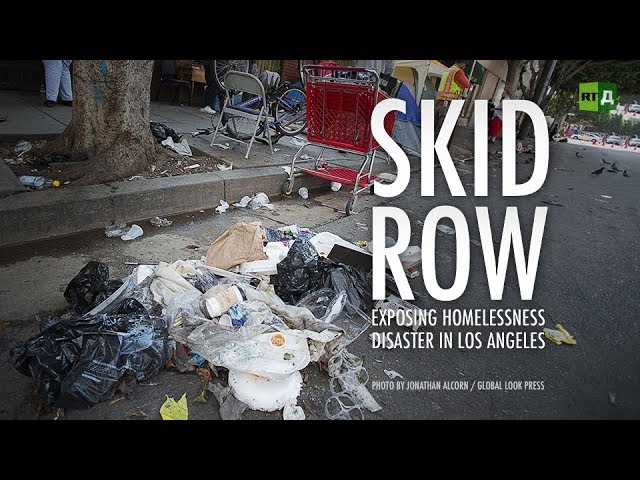The image depicts an extensively littered street on Skid Row in Los Angeles, characterized by the stark and poignant caption in large white capital letters: "Skid Row, Exposing Homelessness Disaster in Los Angeles," with credit to the photographer Jonathan Alcorn from Global Look Press. Dominating the scene is a chaotic assemblage of trash scattered across the gray concrete road and a grimy sidewalk. Among the debris are familiar objects like plastic bags, soda can plastics, coffee cups, an unkempt red shopping cart, an overturned folding chair, and an upside-down bicycle. A trash bag appears to have exploded, spewing its contents—ranging from brown bags to what might be diapers—adding to the disorder.

In the backdrop, a sanitation worker clad in a safety vest appears to be cleaning up, hinting at ongoing but overwhelmed efforts to manage the situation. The base of a tree trunk and the feet and legs of people are also visible, emphasizing human presence amidst the refuse. Birds peck at the litter, adding to the sense of urban decay. A distinctive green RT logo is located in the upper right corner, marking the news organization associated with the image. The photo encapsulates a vivid and distressing snapshot of the dire conditions and pervasive neglect faced by the area, highlighting the severity of the homelessness crisis in this Los Angeles neighborhood.